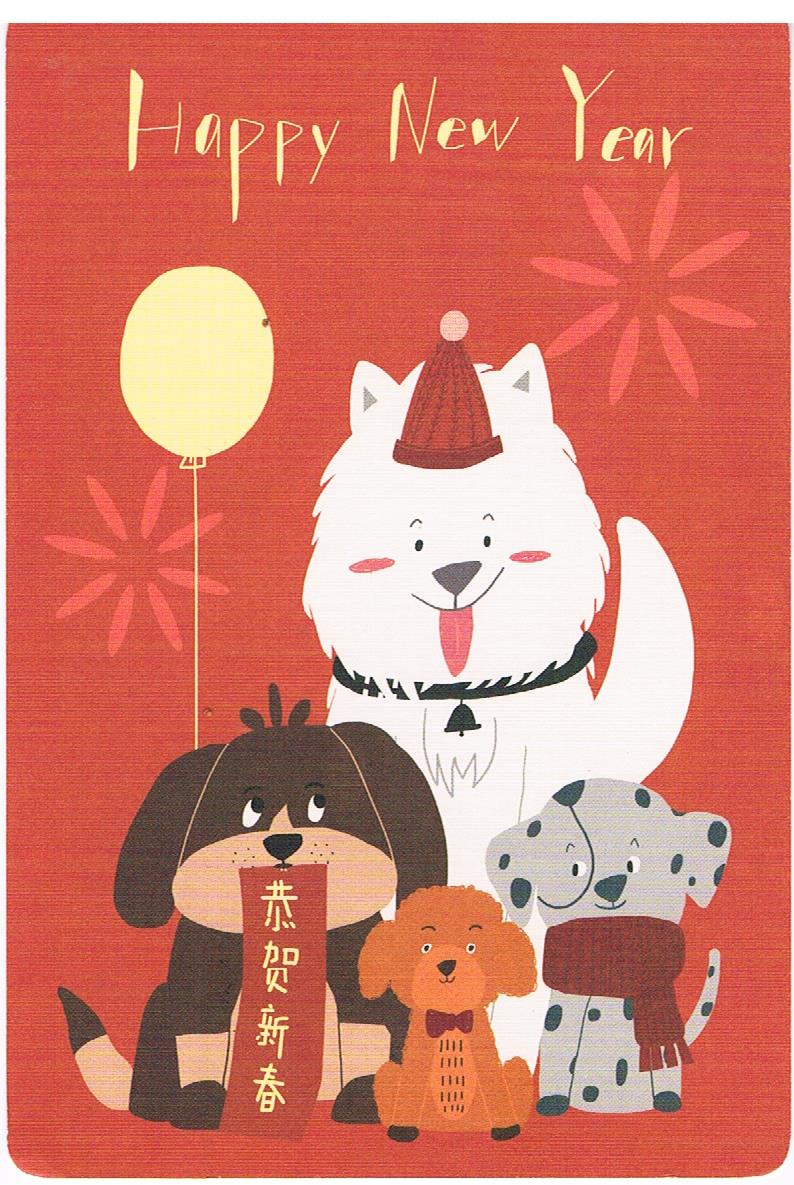This animated New Year greeting card features a vibrant red background with festive elements such as fluttering fireworks and a cheerful yellow balloon. At the top, the message "Happy New Year" is written in playful yellow lettering. The card showcases four adorable animated animals: a brown and peach-colored dog, a large white cat comically sticking its tongue out while wearing a red stocking hat, an orange puppy, and a Dalmatian sporting a red scarf. The orange puppy is shown holding or displaying a sign with Chinese characters, adding a multicultural touch to the celebration. This lively and colorful image is a delightful depiction of a New Year's celebration, blending fun animation with festive spirit.